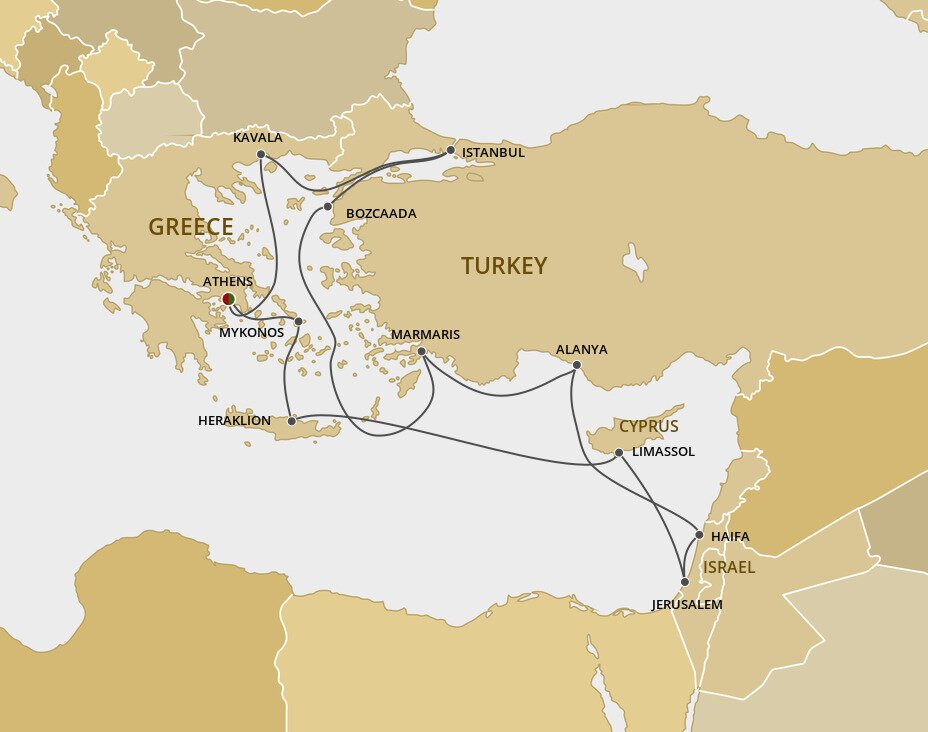This image depicts a simple, digitally-created map of the Mediterranean Sea area and its surrounding countries, including Greece, Turkey, and Israel. The map is colored in predominantly light brown to olive hues, with the Mediterranean Sea in white. Black dots on the map mark key cities such as Athens in Greece, Haifa and Jerusalem in Israel. A series of black lines form a path connecting different countries and cities, likely indicating an expedition, migration, or pilgrimage route. The map is focused on delineating these significant waypoints and routes in this geographic region.